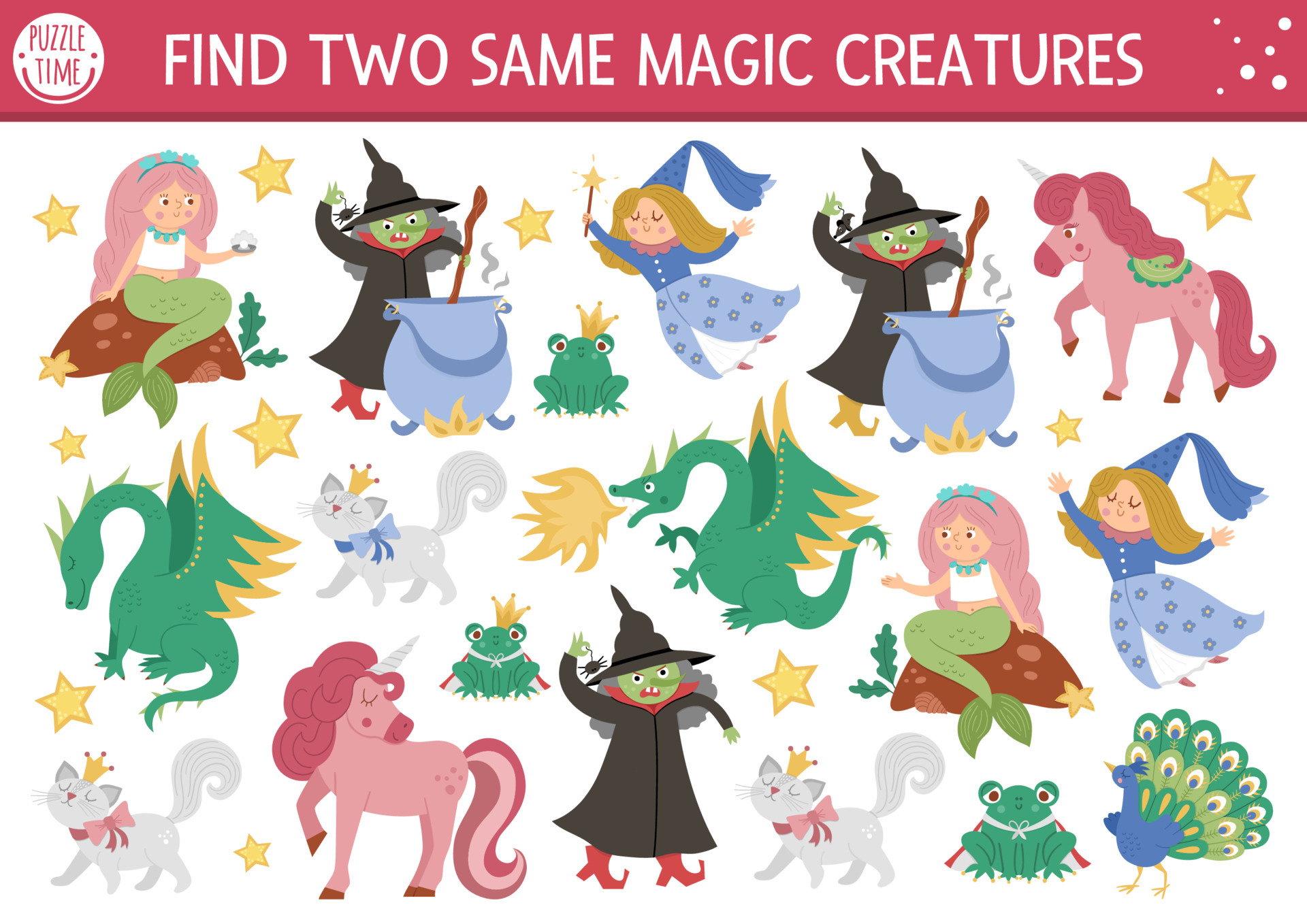The image is a square children's puzzle brimming with vibrant fantasy characters set against a clean white background. Dominating the top of the picture is a pinkish-red banner stretching horizontally from left to right. On the left side of the banner is a small white circle containing the phrase "Puzzle Time" in pink font. Centrally positioned on the banner, in bold, uppercase white letters, is the directive: "FIND TWO SAME MAGIC CREATURES." 

Below the banner, the puzzle displays three rows, each featuring roughly six characters, all presented in a playful, cartoonish style. There's a bounty of magical creatures to find: green dragons with puffy bodies and golden flames, black-robed witches with green faces and silver cauldrons, pink-haired mermaids with green tails, and pink unicorns with flowing manes and white horns. Gray cats adorned with pink ribbons and golden crowns, blue peacocks with vibrant feathers, and green frogs also populate the scene. Scattered gold stars and small white dots add extra sparkle to the playful collage. 

The puzzle invites children to engage by finding matching pairs among the charming lineup of mermaids, witches, unicorns, dragons, cats, frogs, and peacocks.